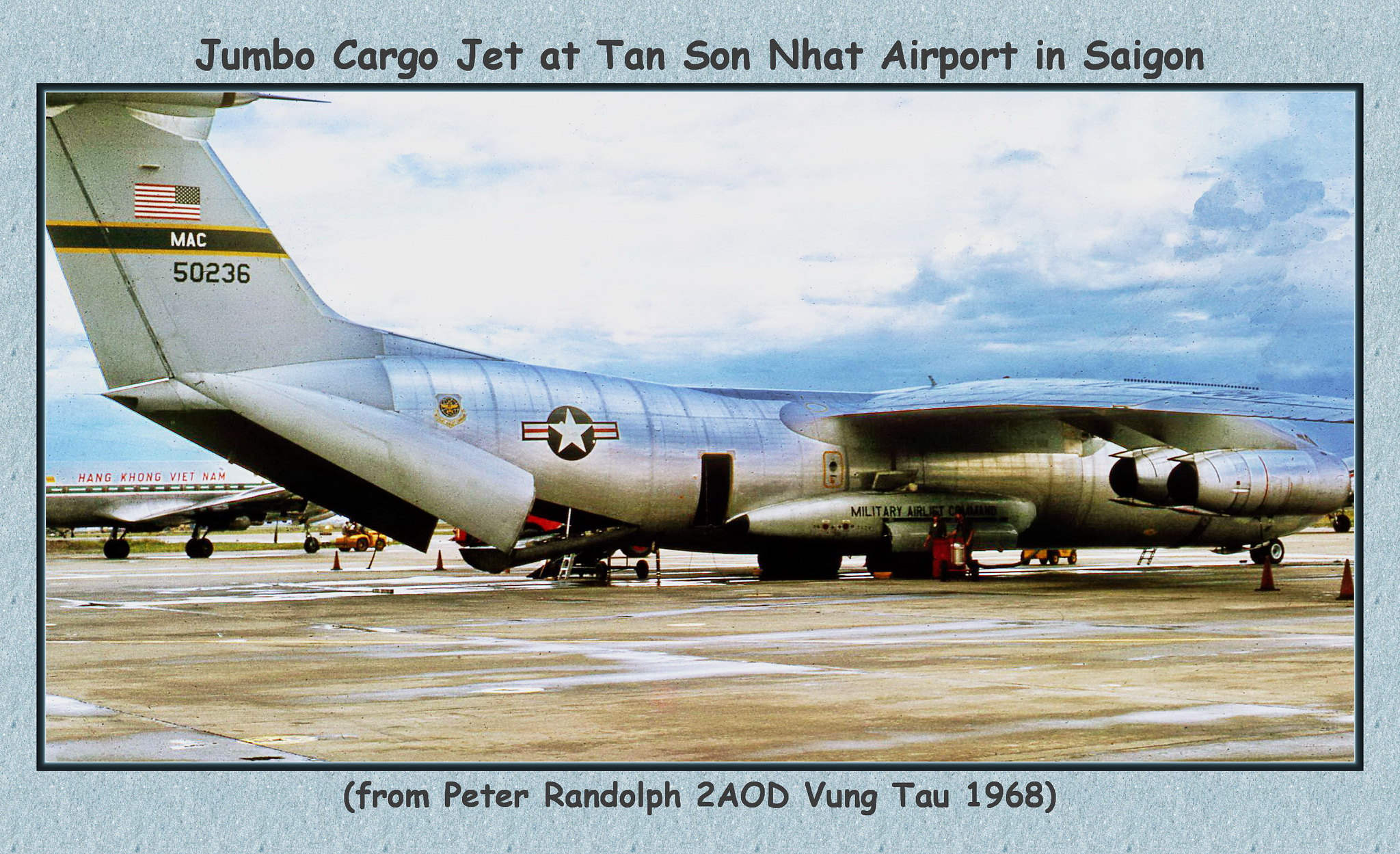The photograph, prominently centered and framed with a light blue matte border, depicts a sizeable silver Jumbo Cargo Jet stationed at Tan Son Nhat Airport in Saigon. The top of the image contains the text "Jumbo Cargo Jet at Tan Son Nhat Airport in Saigon," while the bottom reads "From Peter Randolph to AOD, Vung Tau, 1968." The aircraft, adorned with a United States flag on its tail and a U.S. Air Force logo on its middle section, also bears the identifier "MAC" and the number "50236." The detailed photo reveals a star medallion and a gold eagle emblem along the plane's body, hinting at its military designation with partially visible "Military Airlift Command" text. The scene is set on a concrete tarmac, with visible clouds occupying the sky above. People are seen moving around the jet, possibly refueling it, alongside orange safety cones and hints of another smaller plane in the background marked "Hang Kong Vietnam." The overall setting appears to be an active airport, captured during the daytime in 1968.